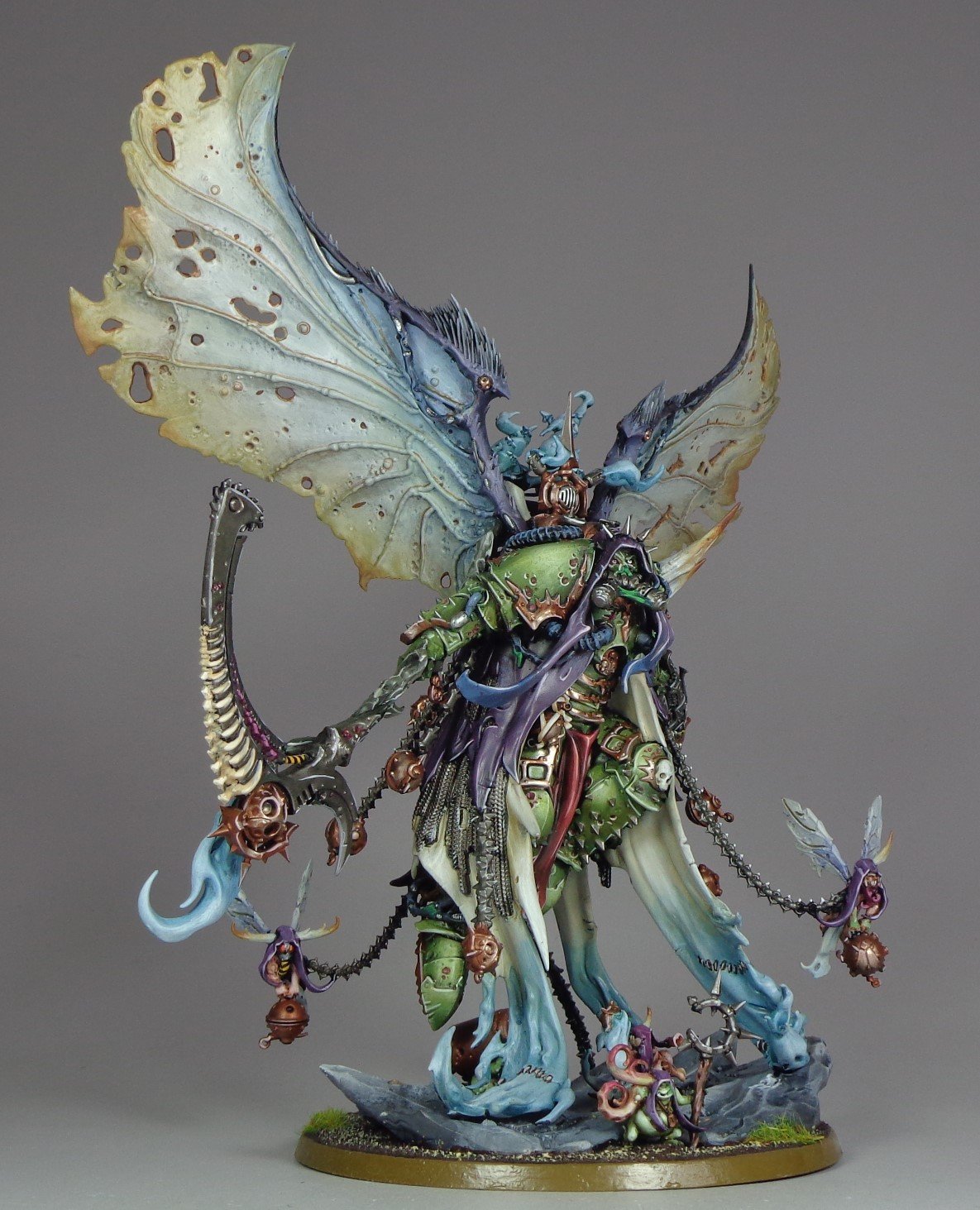This detailed image features an ornate, mystical figurine resembling a combination of a dragon and a fairy, set against a whitish-gray background. The statue stands on a greenish-gold round base and is lavishly decorated with vibrant colors, including greens, blues, reds, whites, and yellows. The creature has large, elaborate wings extending upward from its back, suggesting a dragon or fairy-like appearance. It is adorned in ornate, colorful robes and ribbons, and accessorized with various jewels and dragonflies, enhancing its fantastical aesthetic. The figurine appears to be armored, with chains and weapons, including a spear embedded in the ground featuring a wooden shaft and a spiked "C" shape. Overall, the statue exudes a futuristic and mystical vibe, made from materials that look like metal and plastic.